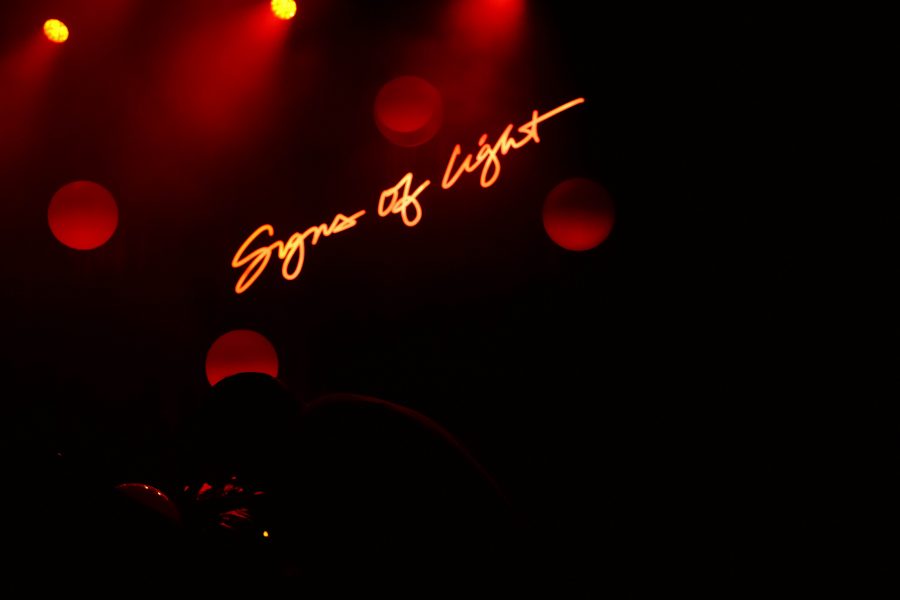The image is a dark, artistic composition meant to evoke emotion and inspiration. The backdrop resembles that of a concert or stadium, bathed in darkness except for two yellow spotlights in the upper left corner, casting a red beam of light downwards into the void. This illumination creates a striking effect, revealing four to five red orbs or bubbles suspended in the air. In the center of the image, a neon cursive font stands out, glowing brightly in a golden-orange hue, spelling out "Signs of Light." This electric sign style text is the focal point amidst the scattered red droplets and the surrounding abyss. There may be a hint of a person bending over at the very bottom of the image, though the darkness obscures this detail, keeping the viewer's attention on the central message.